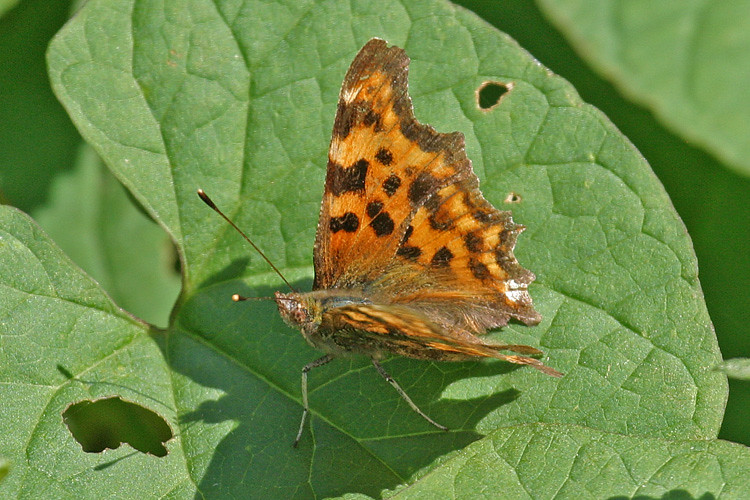In this captivating close-up image taken outdoors, a striking moth or butterfly rests on a large, vibrantly green leaf riddled with insect holes, suggesting previous feedings. The leaf, healthy and unwilted, provides a sturdy perch for the creature. Its wings, primarily a vivid orange adorned with white, leopard-like spots, taper into edges bordered with a deep, near-black brown color. The head of the insect, shaped reminiscently of a fish or angle, features prominently large antennae sprouting from it. Visible are two of its long, segmented legs, while the rest are obscured by its wings. The background showcases blurred foliage, highlighting the focus on the intricate details of the insect and its verdant resting spot.